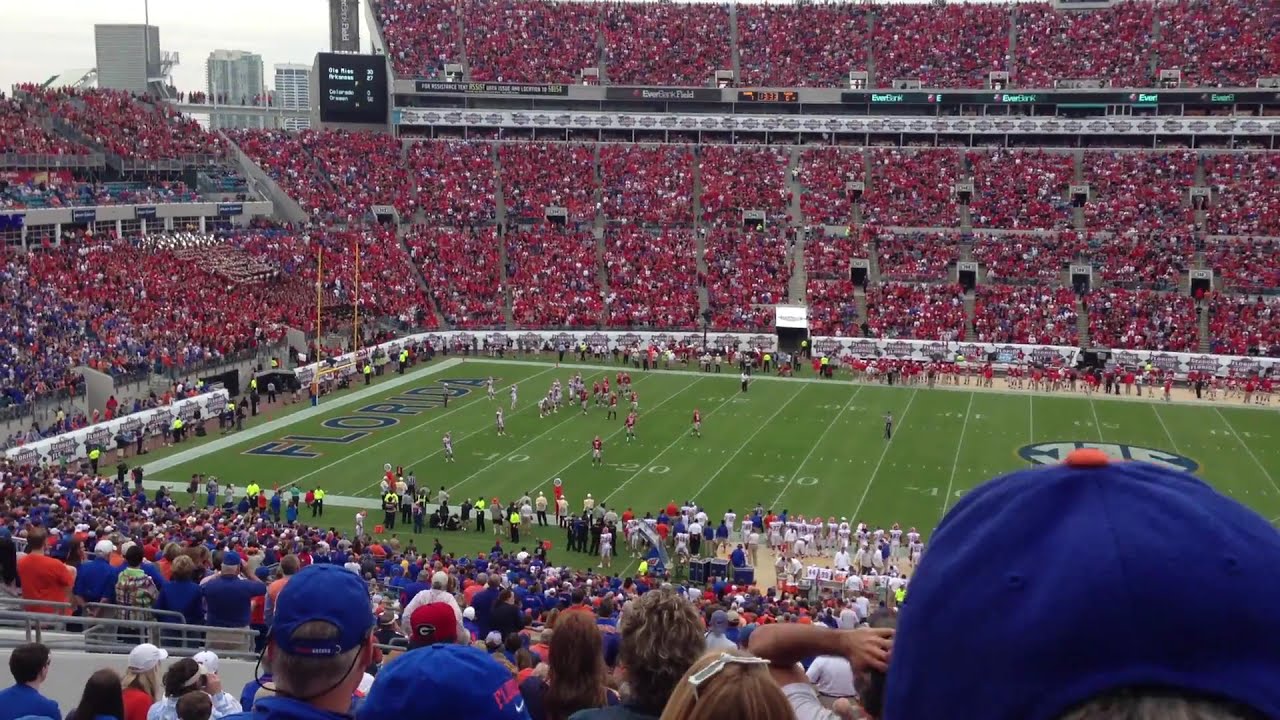This image captures the bustling excitement of a packed football stadium, viewed from a tiered vantage point. Dominating the scene, the three-quarter length field showcases a crucial play-in-progress near the left goalpost, prominently marked with the word "Florida," indicating the University of Florida's home turf. Fans on the far side of the stadium create a sea of red, signifying their allegiance, while those nearer to the camera are adorned in a vibrant mix of blue and orange, the colors of the Florida Gators. On the sideline, officials in neon green shirts stand ready, a visual contrast against the player jerseys. The two teams, one in white and the other in red, are positioned with the red team facing left and the white team facing right, poised for action near the 10-yard line. The atmosphere is punctuated by security staff in neon shirts and a head in a blue baseball cap with an orange dot visible in the bottom right corner, partially obscuring the school's emblem at the center of the field. Above the stadium, an overcast sky looms over tall skyscrapers seen in the upper left, adding a cityscape backdrop to the lively sporting event below.